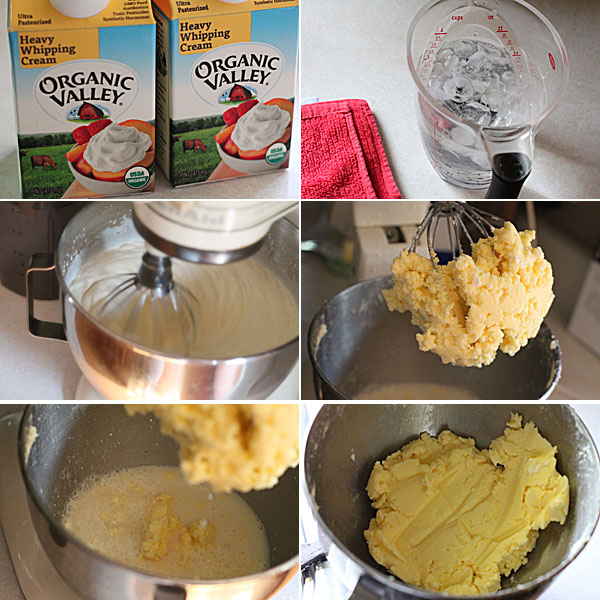This collage showcases a detailed step-by-step process of making a cream-based batter through six meticulously captured images. The sequence begins at the top left corner with two pint cartons of Organic Valley heavy whipping cream. Adjacent to it, on the right, is a measuring cup filled with ice water, partially obscuring a red microfiber cloth. Moving downward, the middle left image features a KitchenAid mixer actively whipping up the batter. The corresponding image to the right illustrates the clumpy batter adhering to the mixer's whisk attachment. In the first image of the bottom row, we observe the whisk attachment pulled out of the mixture, highlighting the thick consistency of the batter, as the liquid components appear to be largely incorporated or evaporated. The final image on the bottom right presents the end product— a dense, yellowish, clumped batter resting in the KitchenAid's stainless steel mixing bowl.